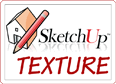The image showcases an intricate layout formed entirely from interlocking, rectangular pieces of wood arranged in zigzag or "W" patterns. These pieces, blending seamlessly in shades of white, beige, and off-white, create a visually striking, left-to-right pattern that spans approximately 40 rows. At the center of the image, there's faint gray text reading "Sketchuptextureclub.com," hinting at its purpose as a background texture for 3D graphics programs. Dominating the middle is a small house topped with a pencil, both rendered in gradient tones of gray and white, further emphasizing the image's detailed craftsmanship and subtle color palette.